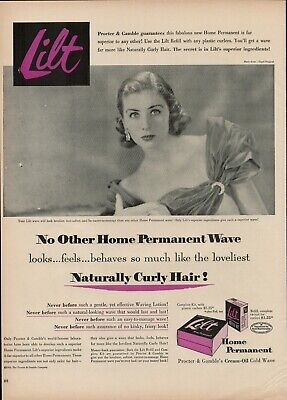This vintage magazine advertisement, likely from the 1930s or 1940s, showcases the Lilt home permanent wave treatment. The ad is predominantly black and white with a touch of purple. A notable black box in the top left corner displays the product name "Lilt" in purple letters. Beneath it, a black-and-white photo of a glamorous woman with a 1920s to 1940s flapper-esque style is featured. Her hair, slicked back with curls at the nape, and off-the-shoulder dress with a pronounced ruffle, exudes classic elegance.

The prominent headline reads, "No other home permanent wave looks, feels, behaves so much like the loveliest naturally curly hair." This slogan underscores the product's promise of delivering natural-looking curls. At the bottom right, there is an image of the Lilt product package, which includes a cream oil treatment, clearly marked by the Procter & Gamble brand. The page is discolored to a sepia tone, hinting at its age and adding to the nostalgic charm. This carefully crafted advertisement captures the allure and sophistication of the period while promoting a beloved hair care solution.